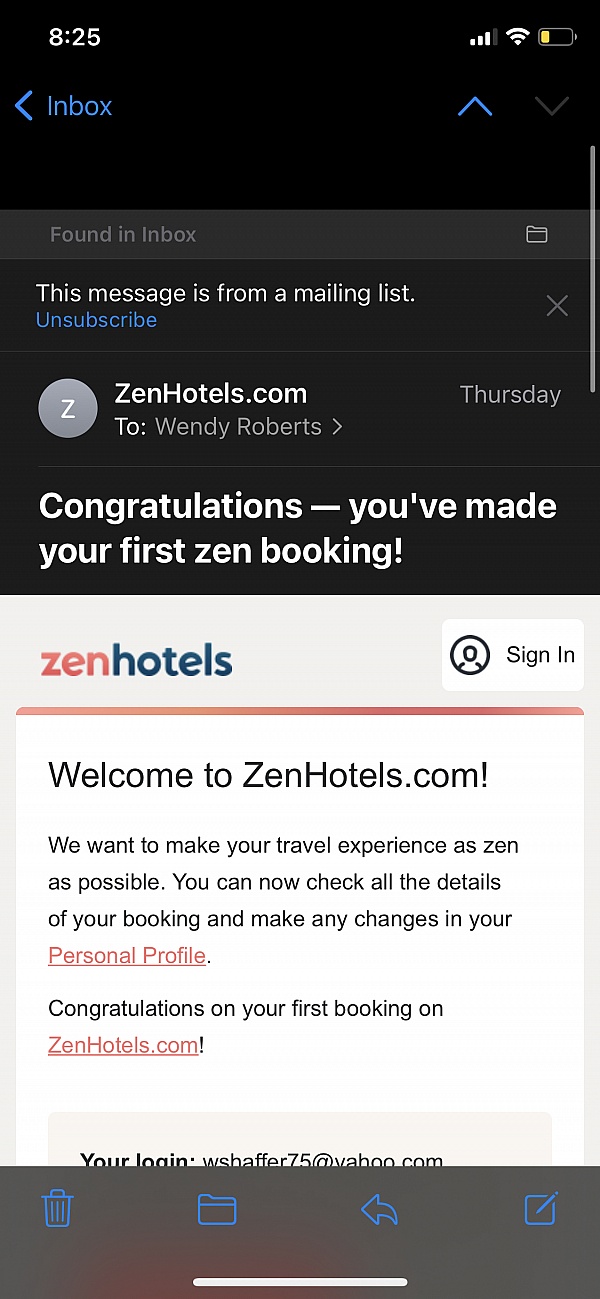The image is a vertically oriented rectangular screenshot of an email interface.

The upper half of the image has a predominantly black background. In the top left corner, "8:25" is displayed in white font, indicating the time. Beneath the time, in turquoise font, the word "Inbox" is accompanied by a left-pointing arrow. On the right side of this section, an icon depicting a battery with a yellow indicator and two arrows—one turquoise pointing up and one gray pointing down—are visible.

Below this, a light black horizontal bar features the text "Found in Inbox" on the left and a small file icon on the right. Underneath this bar, in white font, the message "This message is from a mailing list." is displayed, with an "X" icon to the right and the word "Unsubscribe" in turquoise below it. Adjacent to this, a circle with a white background contains a bold white "Z" in the center. To the left of the circle is the bold white text "zenhotels.com," and on the far right, the word "Thursday" is visible. Beneath this, the email is addressed to "Wendy Roberts," followed by the bold white text "Congratulations. You've made your first zen booking!"

The lower half of the image has a white background. At the top, the text "zenhotels" is in lowercase with "zen" in orange and "hotels" in blue. To the right of this, the word "Sign In" appears. Below this header, an orange line transitions to red from left to right. In bold black font, the text "Welcome to zenhotels.com!" is shown. Following this, additional text reads: "We want to make your travel experience as zen as possible. You can now check all the details of your booking and make any changes in your personal profile." The phrase "personal profile" is highlighted in orange. Another congratulatory message about the user's first booking on zenhotels.com, where "zenhotels.com" is also in orange and appears as a hyperlink, is included.

At the very bottom, the user is prompted with their login details. The footer of the page has another light black section featuring icons for a waste can, a file, an arrow, and a "Create New" label with turquoise icons.